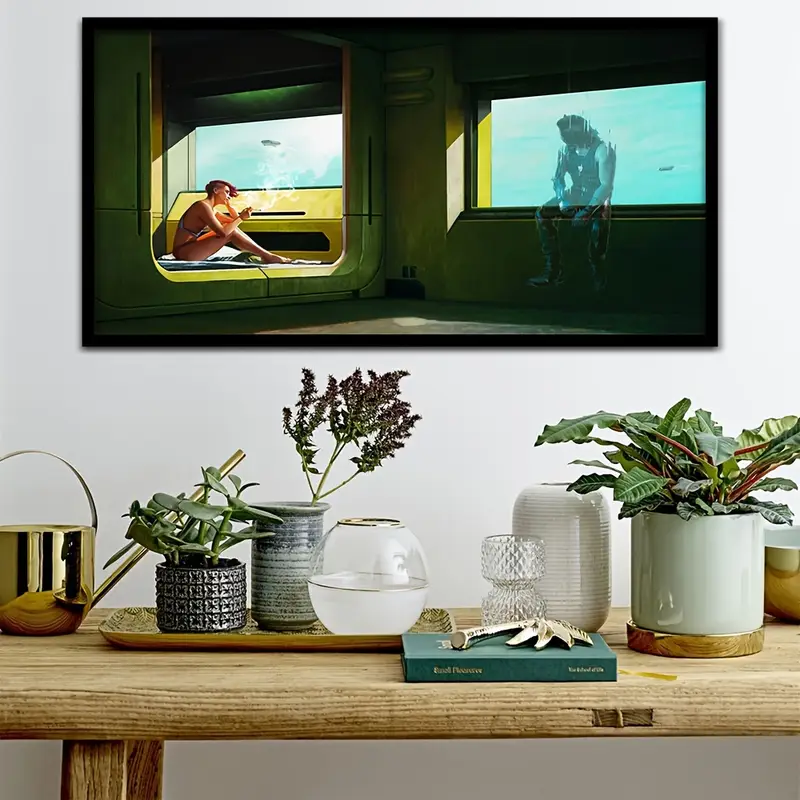In this realistic, square-shaped photograph of what appears to be someone's home, a wooden console table occupies the foreground. Adorning the table are a variety of objects: a bronze kettle, a glass bowl filled with water, and several small vases containing green plants — including a succulent, an herb, and a leafy plant. Also on the table is a green book, partially obscured by a book weight, adding to the eclectic mix of items. Above the table, mounted on a white wall, hangs a framed artwork that exudes a sci-fi aesthetic, reminiscent of Cyberpunk or Blade Runner styles. This digital image is divided into two parts: on the left, a woman appears to be smoking a cigarette, possibly gazing outwards, while on the right, a partially materialized man, akin to a hologram, fades in and out of view. This room scene, probably a living room, intricately combines elements of homey warmth with futuristic art.